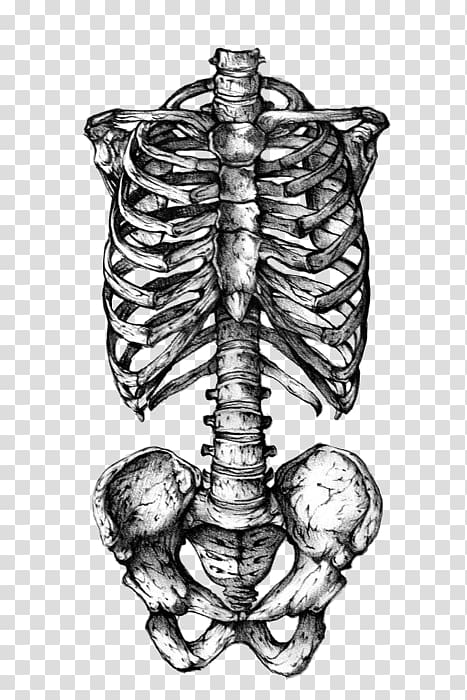This is a highly detailed, black and white pencil drawing of a partial human skeleton. The diagram showcases the rib cage, spine, and hip bones, extending from the neck down to the bottom of the pelvis and spanning to the edges of the shoulders. The spine is depicted from the front, leading down into the tailbone. Notably, there are no muscles or organs present in the illustration; it strictly features the bones. The image is shaded more heavily on the left side of the hip bones, and the background consists of a white and gray checkered pattern. The pelvis appears to have cracks, indicated by black markings. Overall, the drawing is distinct and meticulously rendered.